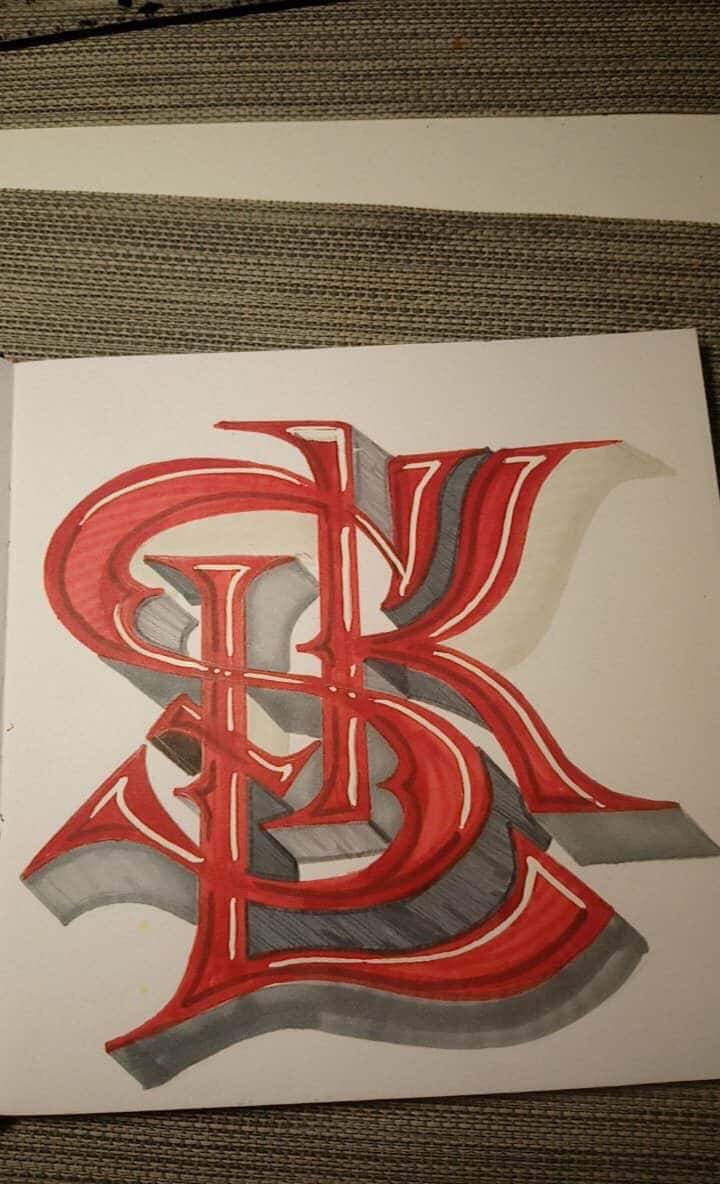This photograph showcases a beautifully hand-drawn piece of art displayed on a white page, likely situated within a sketchbook, which is resting on a white table. Surrounding the paper, you can observe a patterned, textured fabric with horizontal stitches along the top of the image, featuring hues of dark grey and brown, adding a tactile quality to the composition.

The lighting, predominantly emanating from the upper left side, enhances the visibility and details of the artwork. The focal point of the image is a meticulously drawn monogram featuring the letters "S," "K," and "L," artfully rendered in an elegant calligraphy style. These letters are primarily in vivid red, with intricate white highlights to emphasize their form. To create a striking 3D effect, various shades of grey have been skillfully applied, making the letters appear as though they are popping out from the page. This attention to detail and depth demonstrates the artist’s precision and creativity.